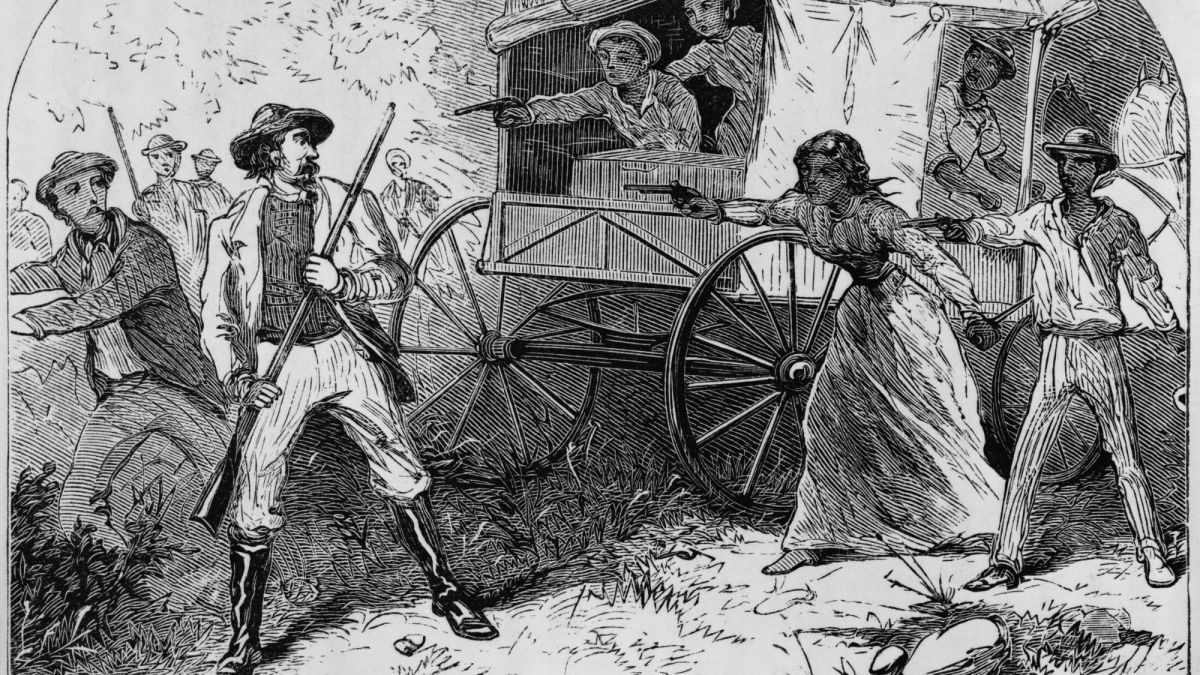The image is a detailed black and white sketch depicting a tense standoff scene likely from the 1800s Wild West. Dominating the right side of the picture is an old-fashioned horse-drawn wagon or carriage. Inside the carriage and standing beside it are four individuals – two seated inside and two adults, a man and a woman, standing on the side. All four are brandishing revolvers, aimed at a group of people to the left. The man beside the carriage is dressed in a jacket with an undershirt, pants, and high black boots, while the woman is clad in a long dress. On the left, a group of men appears to be caught off guard; they hold longer rifles but are not aiming them. The scene is rich with tension, as if an ambush or confrontation is unfolding. The sketch’s monochrome palette of black, white, and shades of gray enhances the historical and dramatic atmosphere.